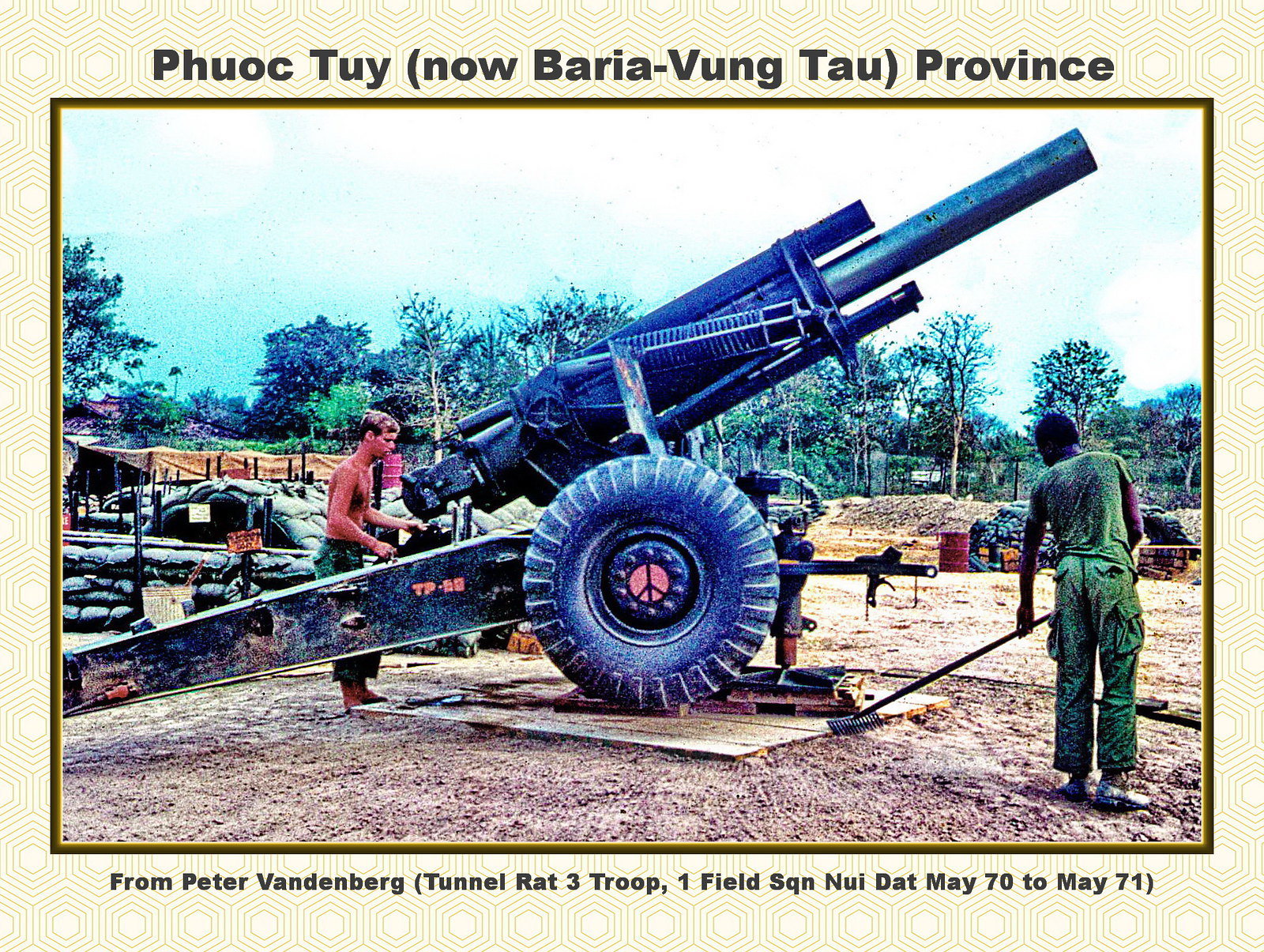This photograph, labeled at the top as "Phuoc Toi, now Baria Vung Tau Province" and captioned at the bottom "From Peter Vandenberg, Tunnel Rep 3 Troop 1 Field SQN, Nui Dat, May '70 to May '71," captures a moment in a military setting in Vietnam. The scene features a large black military cannon with black wheels, amusingly adorned with a pink peace sign at the center of one wheel. The cannon, equipped with a large metal protrusion for stabilization, points towards the upper right corner of the image. In the immediate vicinity, a shirtless Caucasian man in army fatigues operates the cannon from the back, while another individual in fatigues rakes the ground in front of it. The background reveals more military paraphernalia, sandbags, and trees against a partly cloudy sky. The border of the photograph is off-white and gray with a textured appearance. The photo's setting, presumed to be an outdoor military base, is rich with colors including off-white, black, gold, blue, green, brown, pink, and red, capturing the intensity and juxtaposition of war and peace in this vivid scene from Vietnam.